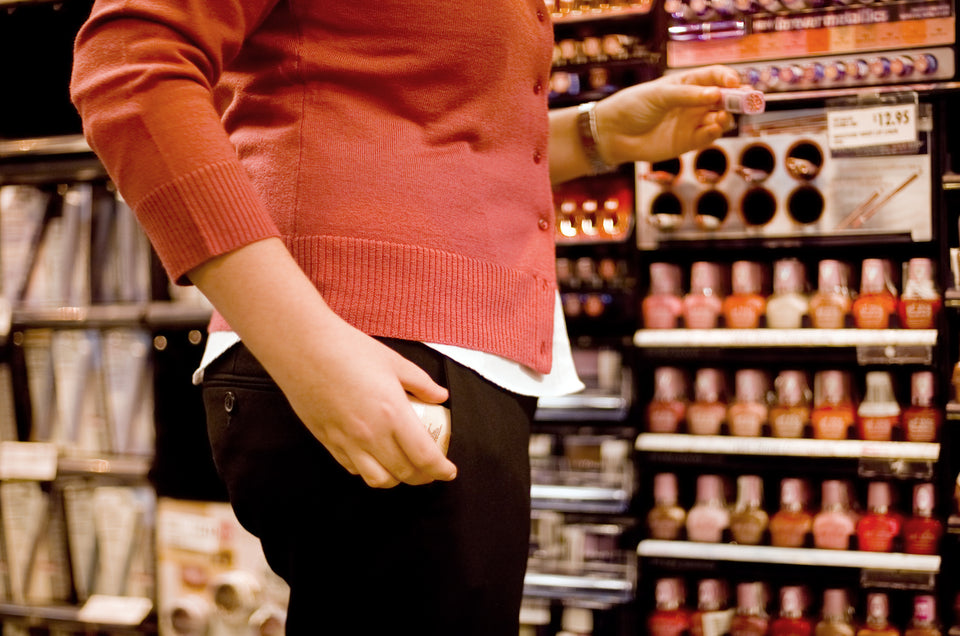In the photograph, a woman is standing inside a store, specifically in the makeup section. She appears to be of fair skin and is dressed in a white shirt layered under a coral-pink button-up cardigan that has orange tones, with black slacks. The sleeves of her cardigan reach about halfway up her forearm, exposing a silver watch on her left wrist. She holds a tube of lipstick in her left hand while her right hand is seen slipping a cream-colored container, possibly face makeup or nail polish, into the pocket of her pants, suggesting she might be shoplifting.

The background of the image features an aisle filled with a variety of makeup products. Directly in front of her are displays of nail polish in various colors. Higher up on the shelves are rows of lipsticks and other makeup items, including what might be eyeliner or eyebrow pencils. The entire scene suggests a makeup department with multiple makeup products organized and displayed on the shelves around her.